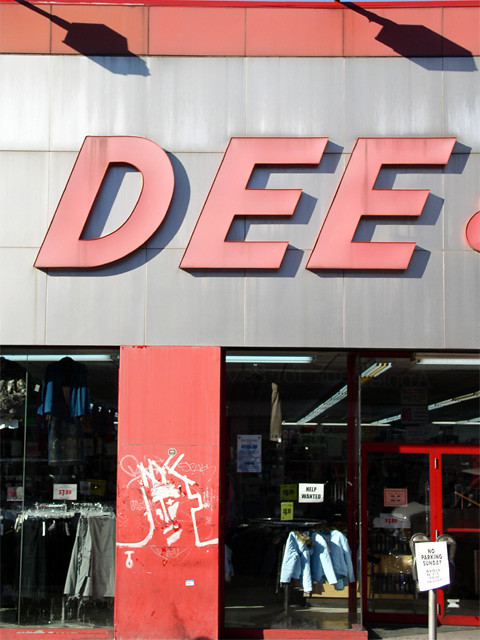This color photograph captures a segment of a storefront. At the top of the image, a partially visible store sign displays the letters "D-E-E" in red against a gray background. Below the sign, several windows showcase the interior of a clothing store, where racks of garments are discernible. On the left side, a rack hangs what may be skirts or pants. A structural supporting beam emerges into view, adorned with white graffiti depicting a schematic image of a man's face. To the right, the probable entryway features glass doors with red frames. Nearby, a small, illegible sign is posted on the walkway outside.